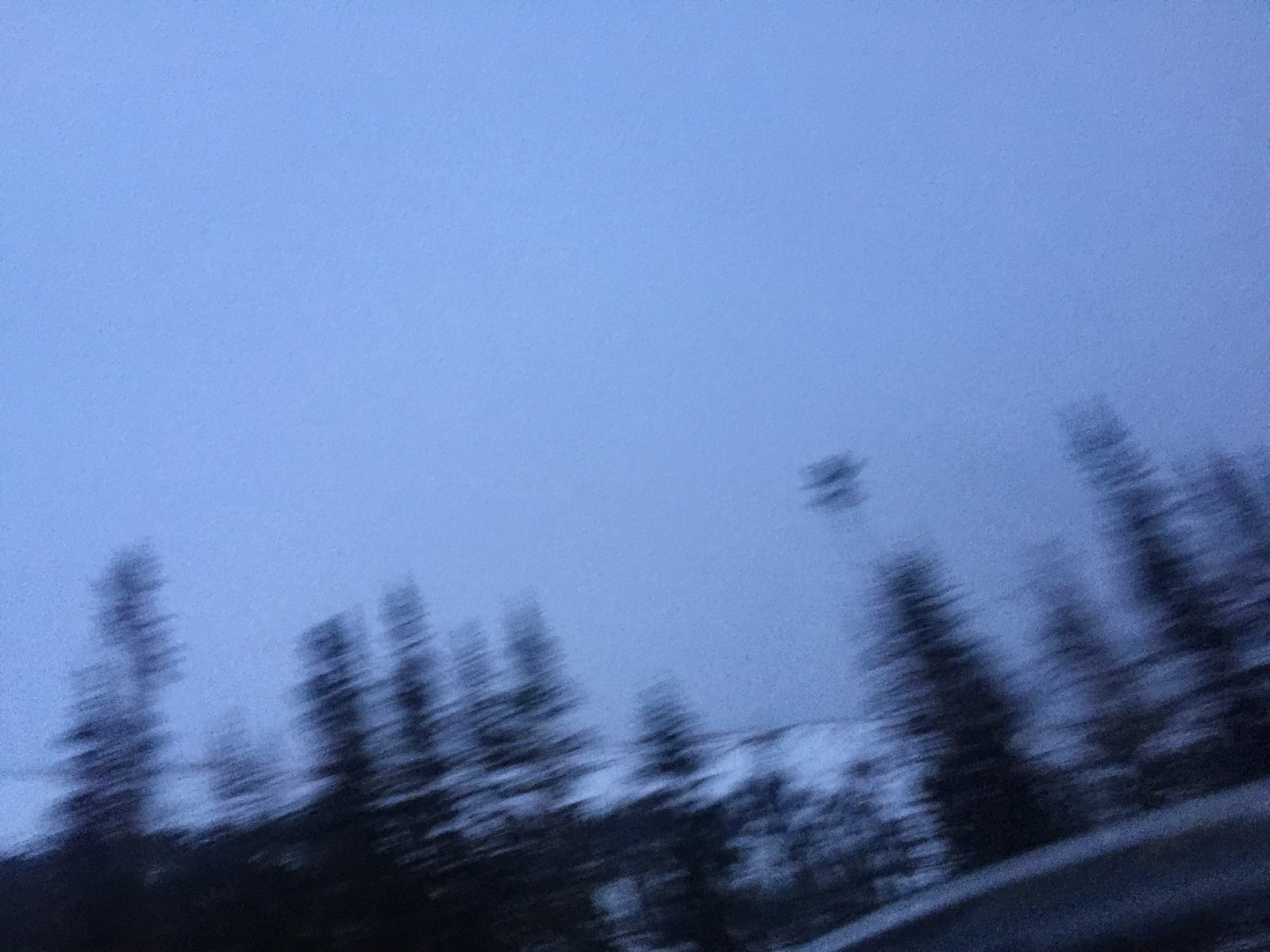This photograph, taken from the perspective of a fast-moving vehicle, captures a dynamic and blurred outdoor scene. The image is shot in landscape orientation and appears to have been taken by someone on the passenger side, possibly holding the camera outside the vehicle. The primary focus is on the sky, which is a light blue hue, indicating a late time of the day with thick cloud cover. Below the sky, dark, tall trees dominate the scene, although they are heavily blurred due to the motion. In the background, there is a faint, blurred impression of a white hill range or snowy mountain, adding depth to the landscape. The bottom right corner of the image reveals part of a silver road barrier, hinting at the road and vehicle presence without showing the street itself. The overall quality and motion blur of the image suggest that the vehicle was moving quickly at the time the photograph was taken, contributing to the dynamic yet unclear capture of the serene landscape.